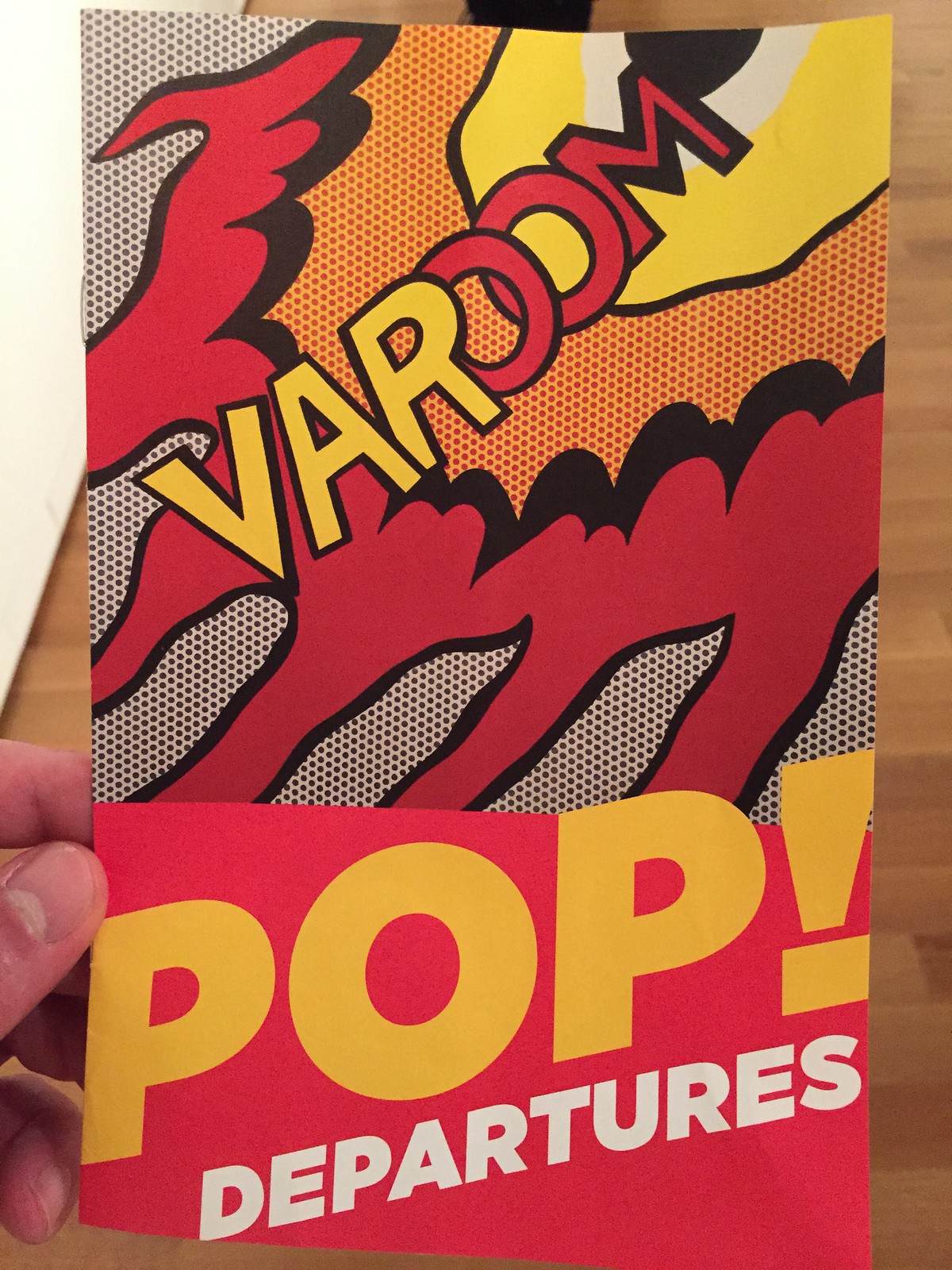This vertically oriented photograph features a vibrantly graphic piece of art with a distinct comic book style. At the top of the artwork, the text "Baroom" is prominently displayed, with "BA" in yellow and "ROOM" in red, surrounded by an explosive burst of colors—black, white, yellow, orange, and red, interspersed with gray specks. Below this dynamic explosion, large letters spell out "POP! Departures" against a plain red background, with "POP!" in yellow and "Departures" in white. A person's hand is visible on the left side, holding up the sheet, with clearly visible thumb and fingers. The background reveals the setting of the photograph, showing a wooden floor and a white wall on either side of the graphic image, indicating the photo was taken in a room with natural lighting.